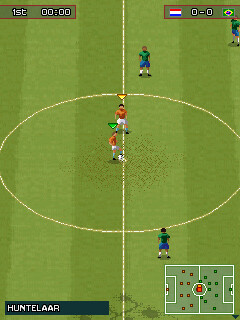The screenshot captures a moment from a pixelated soccer video game. The scene unfolds on a vibrant green astroturf field, adorned with distinct red and yellow markings and a central yellow circle. Two teams face off in vivid pixel art: one team dons red short-sleeved tops and white shorts, whereas the opposing team is clad in dark blue or green t-shirts paired with blue shorts. The team in red currently controls the ball, advancing strategically across the field.

In the upper left corner, the game status is displayed, indicating that it is the first round, accompanied by a visible timer. Adjacent to these indicators, two flags are seen: one with horizontal red, white, and blue stripes, and the other with a green background featuring a yellow diamond and a red center. The score remains at a stalemate, showing 0-0.

In the bottom right corner, a miniaturized version of the soccer field layout is present, serving as a game map to aid players in strategizing their moves. All these elements together create an immersive snapshot of an engaging and colorful retro soccer match in progress.